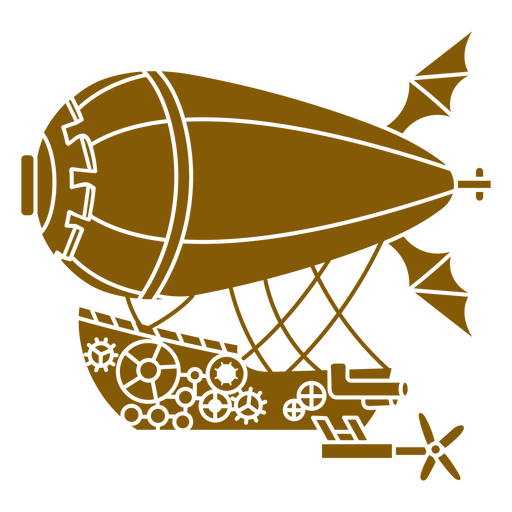The image depicts a detailed, black and white drawing of a unique flying device imagined by an ancient engineer. This contraption features a hot air balloon with two wings and a tail at the back. The balloon is attached by several ropes to a boat suspended underneath. The boat is intricately adorned with mechanical drawings resembling the inner workings of a watch, including numerous cogs and gears. The boat also features a small propeller and an exhaust extending to the back. The entire device showcases a blend of whimsical ingenuity, evoking a sense of flight through mechanical and aeronautical elements.